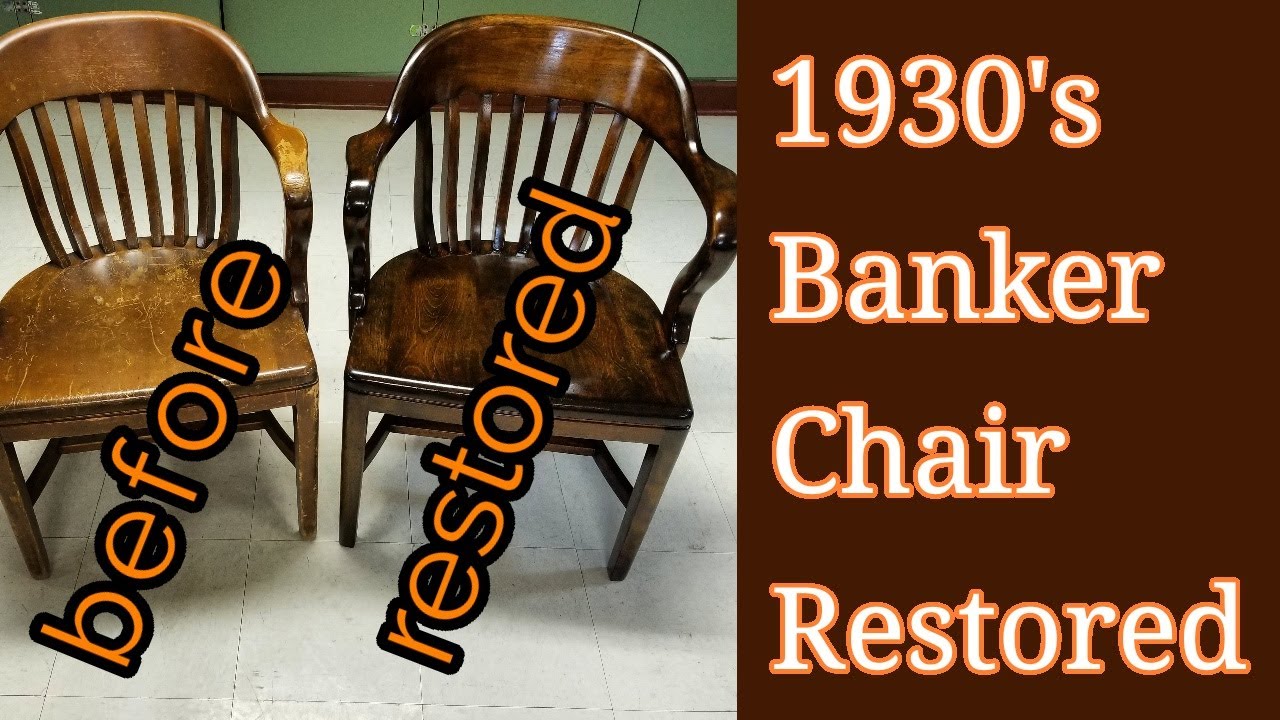The image is a poster showcasing a comparison of two wooden chairs placed in a room with a green wall and light beige tiled floor. On the left side of the image, there are two chairs: the one on the left is a light mocha brown labeled "BEFORE" in yellow-orange font, and the chair on the right is a dark coffee brown labeled "RESTORED" in the same font. Both chairs are wooden with shiny surfaces, featuring round backs with eight vertical poles and two wooden arms. On the right side of the image, against a dark brown rectangular background, cream-colored text framed in orange reads "1930s Banker Chair Restored."